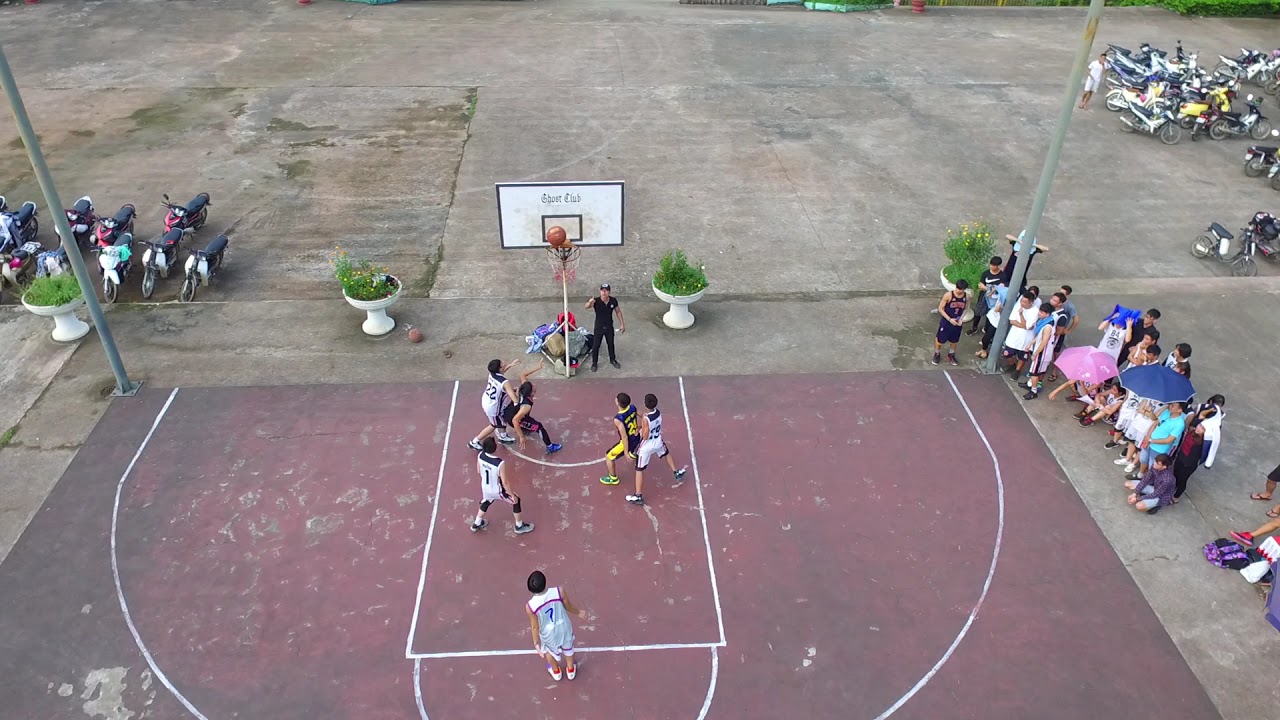The photograph captures an outdoor basketball game on a rust-colored cement court, where six players are in action. Four players wear white uniforms, and two are dressed in blue and gold. The focus is on the basketball as it appears to be going through the hoop, with a man in all black, presumably the referee, standing beneath it. The game's setting is an organized yet informal environment, marked by the presence of spectators to the right, some of whom are holding umbrellas, and a collection of motorcycles or mopeds parked on the left and upper right corners of the image. In the background, behind the hoop, you can see large planters filled with green plants. The white backboard features black lettering, though it is somewhat blurry. The scene is brightly lit by natural daylight, adding to the vivid atmosphere of the game.